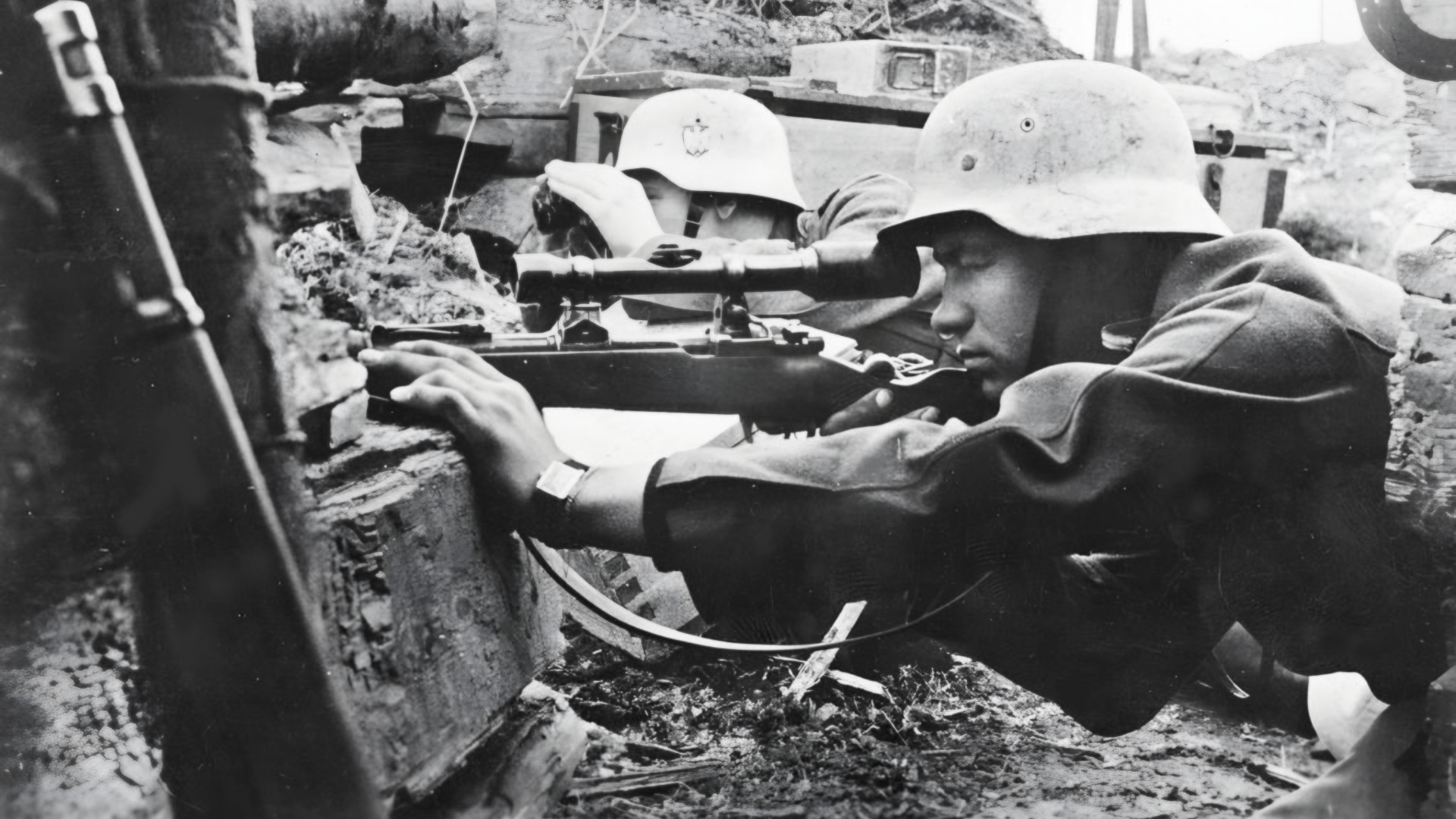This black-and-white photograph, likely from World War I, captures a tense moment in a military trench. Two young soldiers, possibly in their early twenties, are seen wearing light-colored helmets. The soldier in the foreground is intensely looking through the scope of a rifle, while his comrade behind him scans the horizon with binoculars. The trench, marked by dirt and concrete slabs, forms a close-quarters backdrop, and another rifle leans against the short wall behind them. This evocative image highlights the stress and danger of trench warfare, with a mountainous landscape faintly visible in the background.